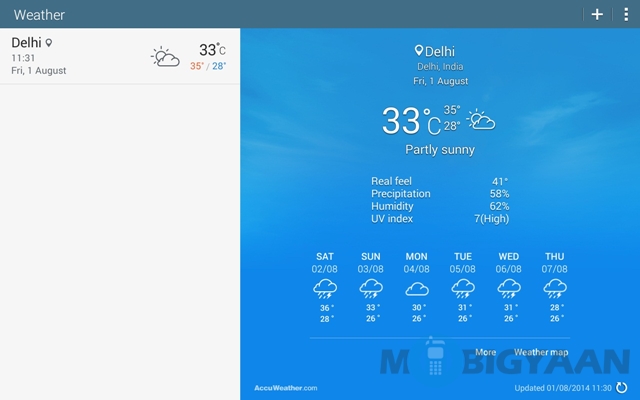### Detailed Weather App Screenshot Description

In the image, we have a comprehensive screenshot taken from a weather application or website. At the very top is a horizontal bar with a blue-grayish hue. On the left-hand side of this bar, "Weather" is prominently displayed in white print, while on the right-hand side, there are two icons: a plus sign and a menu icon.

Beneath this, the location is specified as Delhi. The current time and date are shown as 11:31 on Friday, the 1st of August. Accompanying this information is a partly cloudy symbol, depicting the sun partially obscured by a cloud. The current temperature reads as 33°C. Further down, the forecast details a high of 35°C and a low of 28°C.

To the right side of this primary data, a larger view of the forecast details is visible against a backdrop of a lightly clouded sky. Here it reiterates: "Delhi, Delhi, India," followed by the date "Friday, 1 August" with a current temperature of "33°C," a high of "35°C," and a low of "28°C." The partly cloudy symbol is displayed once again.

Below this section, additional weather details are provided:
- **Partly Sunny**
- **Real Feel:** 41°C
- **Precipitation:** 58%
- **Humidity:** 62%
- **UV Index:** 7 (High)

Across the bottom of the image, the daily forecast is presented in a horizontal layout:
- **Saturday, 2 August:** Thunderstorm symbol, high of 36°C, low of 28°C.
- **Sunday, 3 August:** Thunderstorm symbol, high of 33°C, low of 26°C.
- **Monday, 4 August:** Cloudy symbol, high of 30°C, low of 26°C.
- **Tuesday, 5 August:** Thunderstorm symbol, high of 31°C, low of 26°C.
- **Wednesday, 6 August:** Thunderstorm symbol, high of 31°C, low of 26°C.
- **Thursday, 7 August:** Thunderstorm symbol, high of 28°C, low of 26°C.